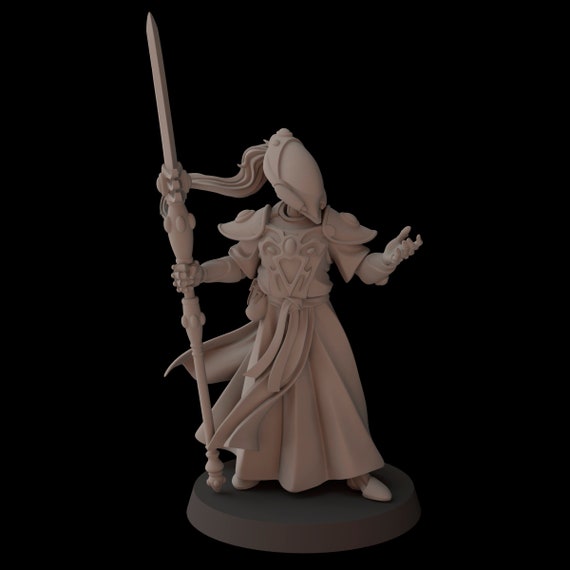This is a highly detailed 3D rendering of a figure with a warm gray hue, lacking any texture or color. The figure stands poised on a dark gray circular platform set against a stark black background. The character is depicted as a person brandishing a long, stylized spear or sword in their right hand, facing the viewer directly, although their head is turned to the right. Their left arm is extended outward with the palm facing up, creating a dynamic pose.

The figure's face is obscured by a mask, but their hairstyle, a ponytail or updo, is shown blowing dramatically behind them. They are clad in armor covering their hands, shoulders, and torso, suggesting a warrior or combatant. The bottom half of the figure’s attire consists of loose, flowing fabric, secured at the waist by visible belt straps, with the fabric and hair both flowing in the same direction, emphasizing a sense of motion.